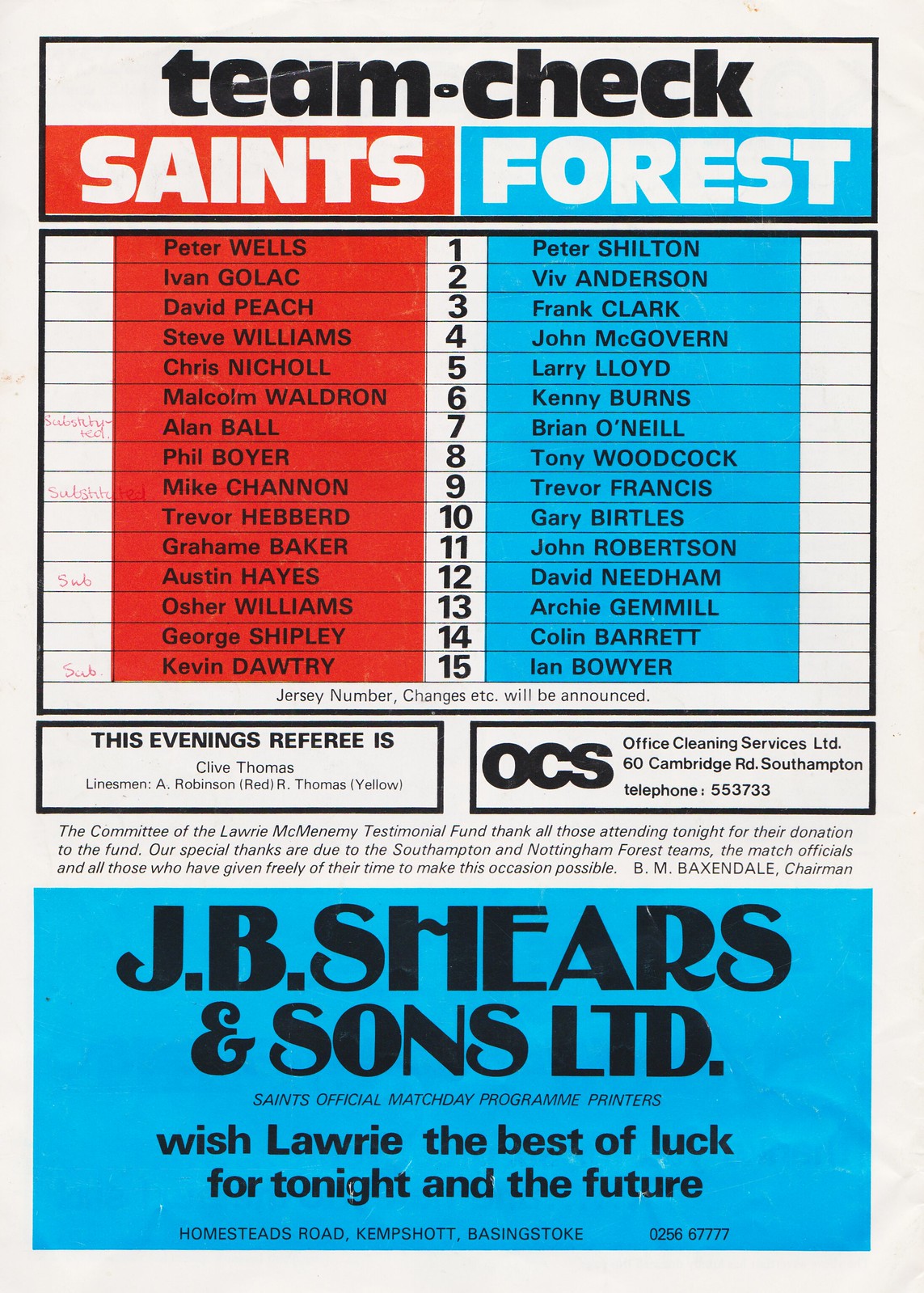The flyer is a detailed team check for a football match between the Saints and Forest, prominently featuring red and blue color themes. On the left side, a vibrant red column lists the Saints players, starting with Peter Wells and includes names like Ivan Golak, David Peach, and Steve Williams, among others, totaling 15 names. On the right, a bright blue column lists the Forest players, starting with Peter Shilton and includes names like Viv Anderson, Frank Clark, and John McGovern, also totaling 15 names. The title at the top reads "Team Check: Saints vs. Forest," showcasing the team colors and respective players prominently. Acknowledgments from the committee of the Laurie McMenemy Testimonial Fund express gratitude to Southampton and Nottingham Forest teams, match officials, and contributors. Sponsors including J.B. Shears and Sons Limited and OCS (Office Cleaning Services Limited) are mentioned, with personal good luck wishes to Laurie from J.B. Shears and Sons Limited. Referee Clive Thomas's name is also highlighted, underlining the official nature of the event. The flyer combines vibrant visuals with detailed informational content, serving both as an advertisement and a heartfelt thank-you message.